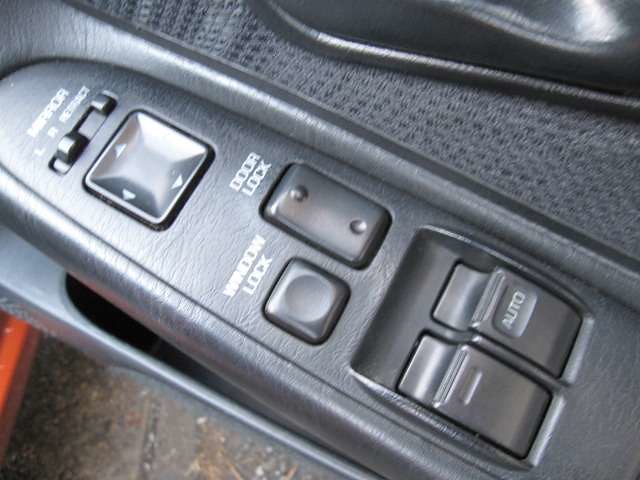This image showcases the interior of a car, specifically the console of the driver side door, assuming the car is designed for right-hand driving. The console is set into black faux leather and features an array of control buttons. At the top, there is a mirror adjustment button that can be slid left and right. Below this is a square button with an indent and an arrow pointing in four directions. To the left of this button is a smaller square button, which operates the window lock function. Adjacent to the window lock button is a rectangular button labeled "door lock" with both indent and out indent designs. Further down, the console includes two window roller buttons. On the opposite side, part of a leather seat with some netting is visible, indicating that the car might be of an older model. The floor on the driver’s side appears somewhat bare and rusted, further suggesting its age.